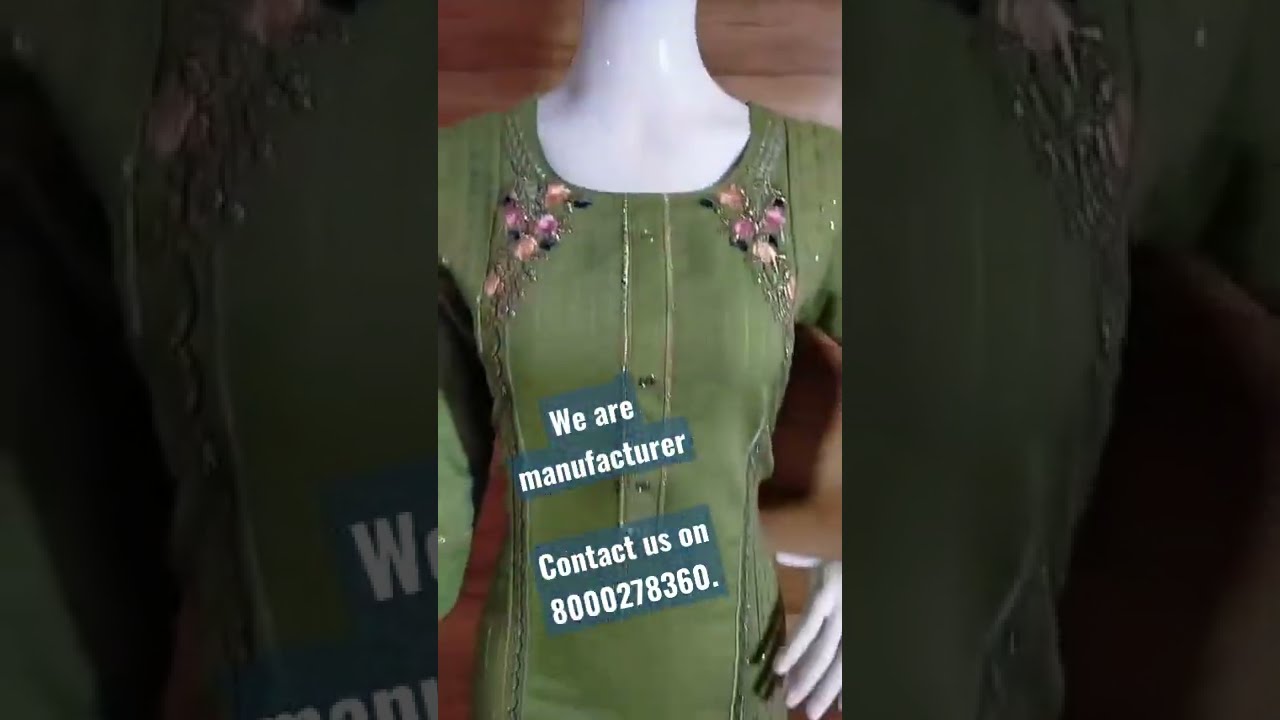In this Instagram-worthy post from a fashion manufacturer, a white mannequin, gracefully standing with its left hand on its hip, showcases an exquisite green dress. The dress, in a sophisticated old-world solid green, features delicate floral accents in pink and white around the collarbone area. Gold accents adorn the collar and trace the line of dark green or black buttons down the front. The sides of the image are artistically blacked-out or grayed-out, focusing attention on the central figure. Overlaying the image, white text on a gray background proclaims, "We are the manufacturer," alongside a contact number, 800-027-8360. The caption reinforces the craftsmanship and elegance of the design, inviting interested patrons to reach out.